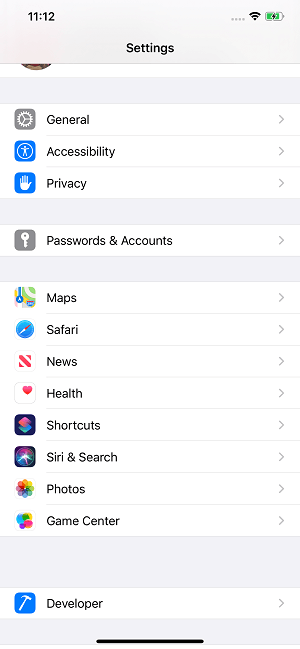This image is a detailed screenshot from a mobile device, specifically an iPhone, displaying a section of the "Settings" menu. The top portion of the screenshot features the status bar, which shows the time as 11:12 in the upper left corner. On the right side of the status bar, the Wi-Fi icon is completely filled, indicating a strong connection, and the battery icon is nearly full. A lightning bolt within the battery icon signifies that the device is plugged in and currently charging.

The main content of the screenshot is centered around the iPhone's "Settings" menu, which is organized in a scrollable list format. At the top, the title "Settings" is positioned slightly below the status bar and centrally aligned on the screen. The settings menu displays various categories, each accompanied by an icon on the left side.

Starting from the top, the first category is "General," represented by a gray gear icon. Below it, "Accessibility" is marked by a blue icon featuring a person silhouette. Next, "Privacy" is indicated by a blue icon with a white handprint. Following that is "Passwords & Accounts," denoted by a gray icon displaying a white key.

The remaining categories continue in the following order:
- "Maps" 
- "Safari" 
- "News" 
- "Health" 
- "Shortcuts" 
- "Siri & Search" 
- "Photos" 
- "Game Center" 
- "Developer"

Each category is listed with its respective icon, providing a visual cue next to each setting option. The screenshot captures the clean and organized interface typical of an iPhone's settings menu.